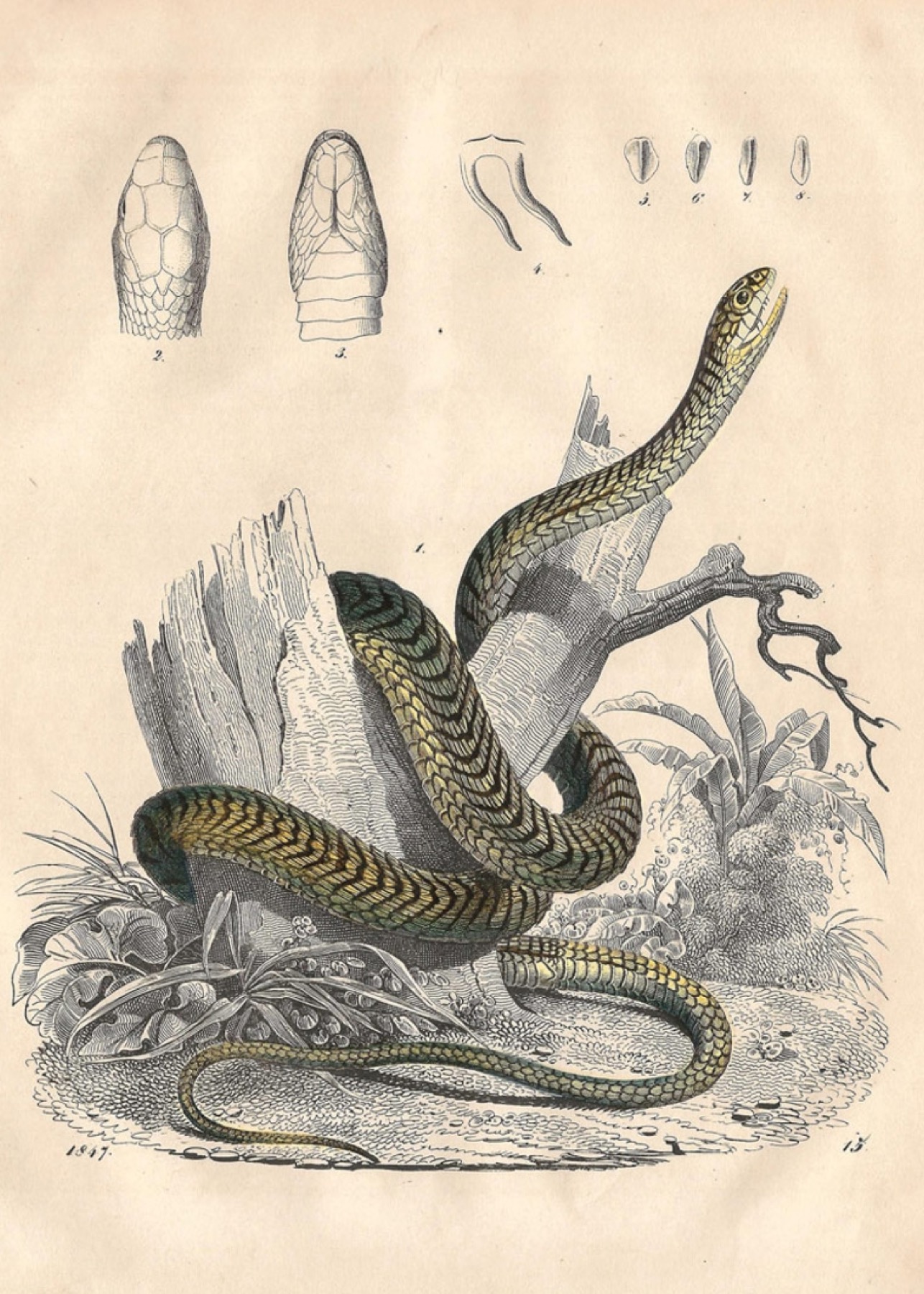The illustration, drawn on an off-white, beige piece of paper resembling aged maps, presents a detailed depiction of a snake intertwined around the trunk of a tree. The snake, the only colored element in the picture, is rendered in rich greens and browns, contrasting with the black and white pencil drawings of the tree trunk, which is broken and surrounded by grass and elaborate fern-like leaves. In the background, additional plants and trees are drawn in grayscale, enhancing the detailed natural setting. 

At the top of the image, a meticulously crafted diagram showcases various views of the snake's head, including a frontal and underside perspective revealing its fangs, as well as detailed sketches of its scales and tail tip. The diagram consists of four parts, each providing clear, intricate insights into the snake's anatomy. Small, faint script at the bottom of the paper reads "18, 47, 15," adding an enigmatic detail to the antique-like drawing.